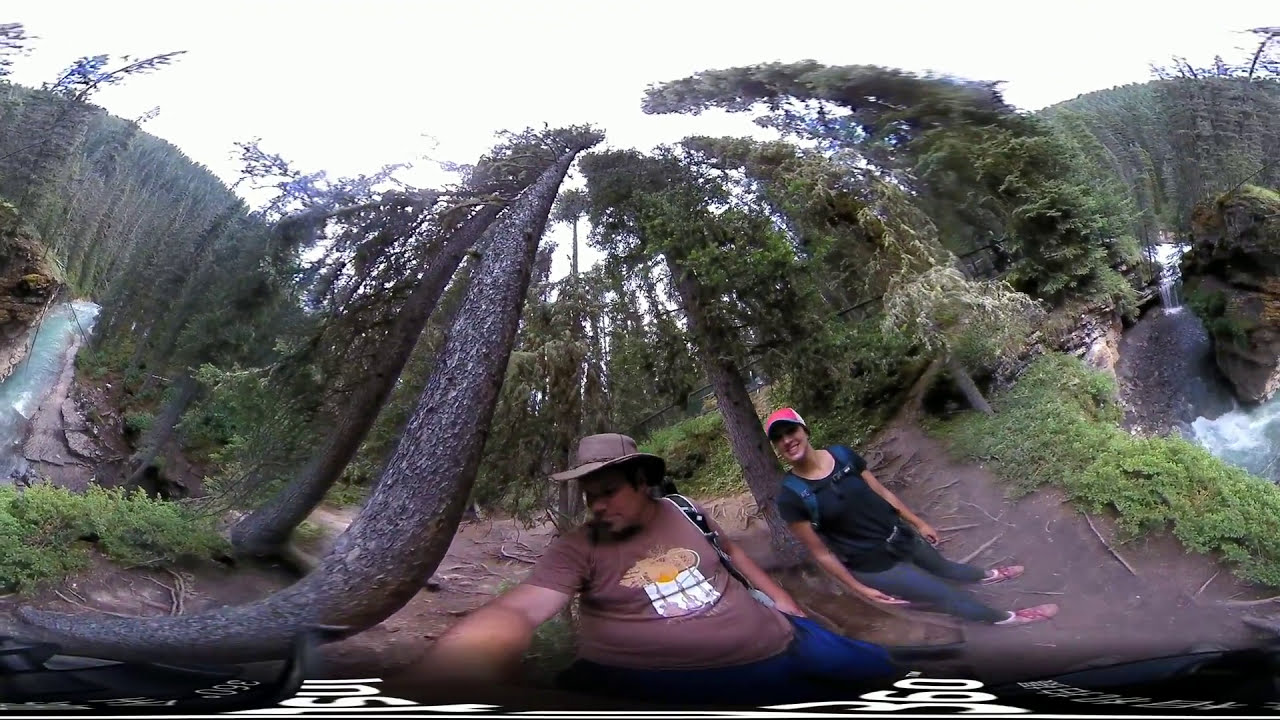In the distorted selfie image, two hikers are centered at the bottom, framed by tall, curved trees. The man on the left, who has tanned skin, a dark goatee, and is wearing an Indiana Jones-style brown hat and graphic brown t-shirt, appears to be taking the photo. He carries a backpack with light blue straps. The woman beside him has pale skin, a red baseball cap, a black short-sleeved shirt, and gray pants, and she is also wearing a backpack. Their surroundings are a lush forest with green-leaved trees that have grayish trunks. To the right of them runs a light blue river with visible rapids, bordered by a large rock formation in its center. To the left is another part of the river flanked by higher rocks and more distant trees. The image, likely taken in a forest or natural area during a hike, is heavily distorted, particularly at the edges, making the trees curve dramatically inward like an elephant's tusk.